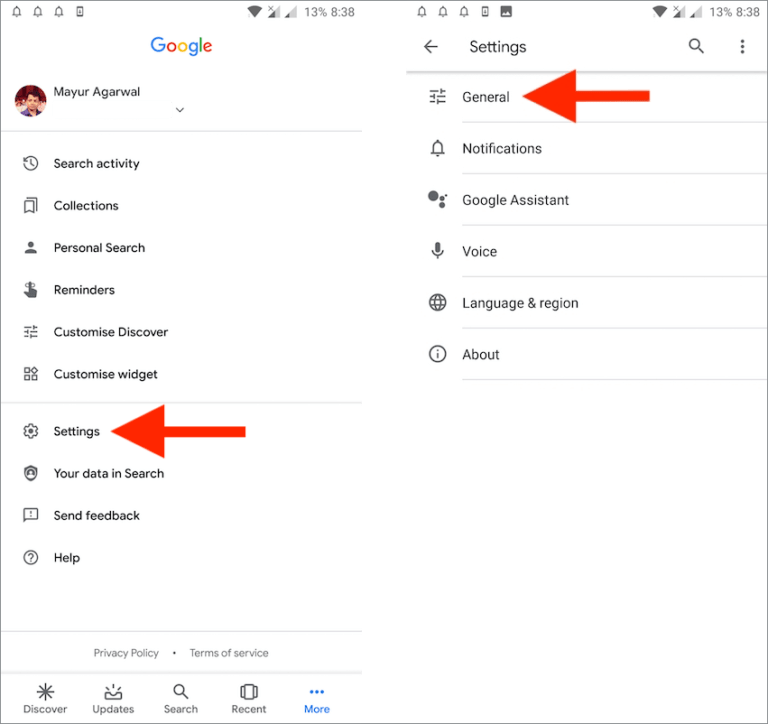The image depicts two overlapping side-by-side screenshots on a smartphone, giving the illusion of a single screen. The left screenshot displays the Google Settings menu with the Google logo at the top-left corner. Below the logo, the user’s profile photo and name, "Meyer Agarwal," are visible. The menu items listed include Search Activity, Collections, Personal Search, Reminders, Customize Discover, Customize Widgets, Settings, Your Data in Search, Send Feedback, and Help. The Settings option is highlighted with a large red arrow pointing towards it. At the bottom, the Discover, Update, Search, and Recent options are faintly visible.

The right screenshot zooms in on the Settings menu with the "General" option highlighted by a red arrow. The subsequent menu items include General, Notifications, Google Assistant, Voice, Language, Region, and About. Each menu item has a light gray icon to its left, against a white background.

Overall, the image provides a detailed view of the Google Settings interface on a smartphone, complete with user profile details, various menu options, and navigational cues highlighted with red arrows.